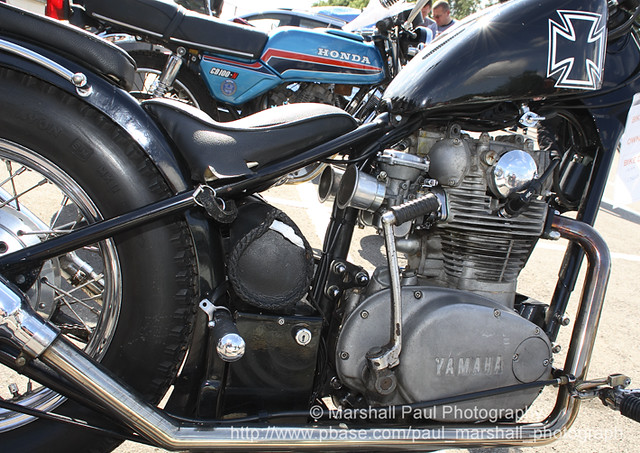In this detailed image, we find ourselves outdoors on a bright sunny day, focused on a black Yamaha motorcycle. The close-up centers on the engine and rear wheel section, revealing an intricately detailed Yamaha engine surrounded by silver aluminum tubing and a big black wheel. To the left, the rear wheel's center is visible, transitioning right towards the seat and stopping short of the handlebars, leaving the front wheel out of frame. 

A prominent black cross with a white outline is visible on the front body of the motorcycle. The background features a light blue Honda motorcycle, adorned with white text across its front body and accented by red and black stripes. The seat and saddle of the Honda are black, and the scene includes pedestrians in the background, observing the motorcycles. The bottom right corner signifies the credit to Marshall Paul Photography, with a URL http://www.pbase.com.